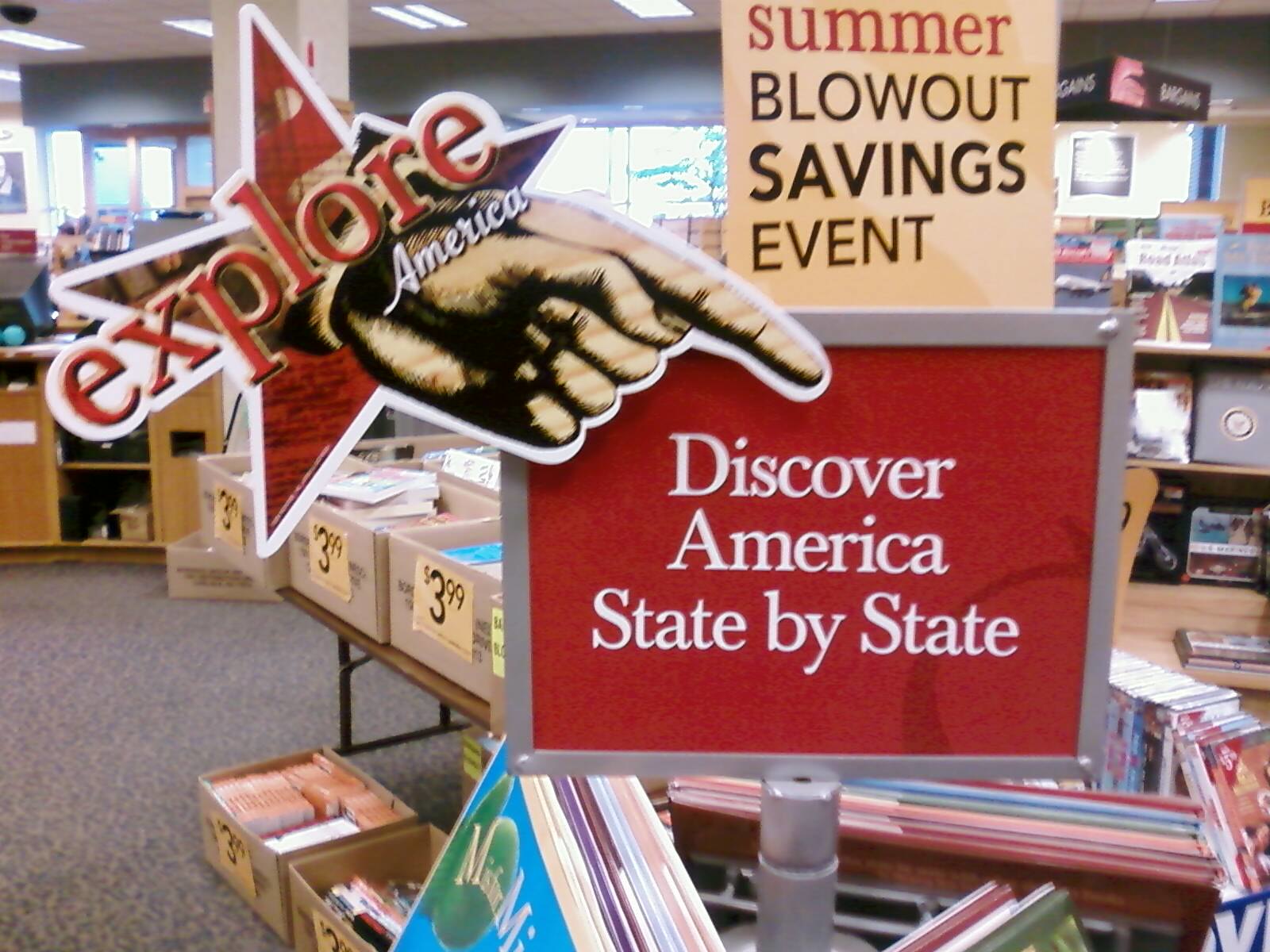In this photograph of a bookstore interior, we observe several racks filled with various books, though the titles are out of focus and difficult to discern. In the foreground, a sale area is prominently featured, displaying multiple boxes of books arranged on tables, each marked with a price tag of $3.99. A striking red sign at the front reads "Discover America State by State" and is adorned with a large cardboard hand inscribed with "Explore America." Above this, a substantial beige sign announces a "Summer Blowout Savings Event," emphasizing the promotional nature of this section within the bookstore.